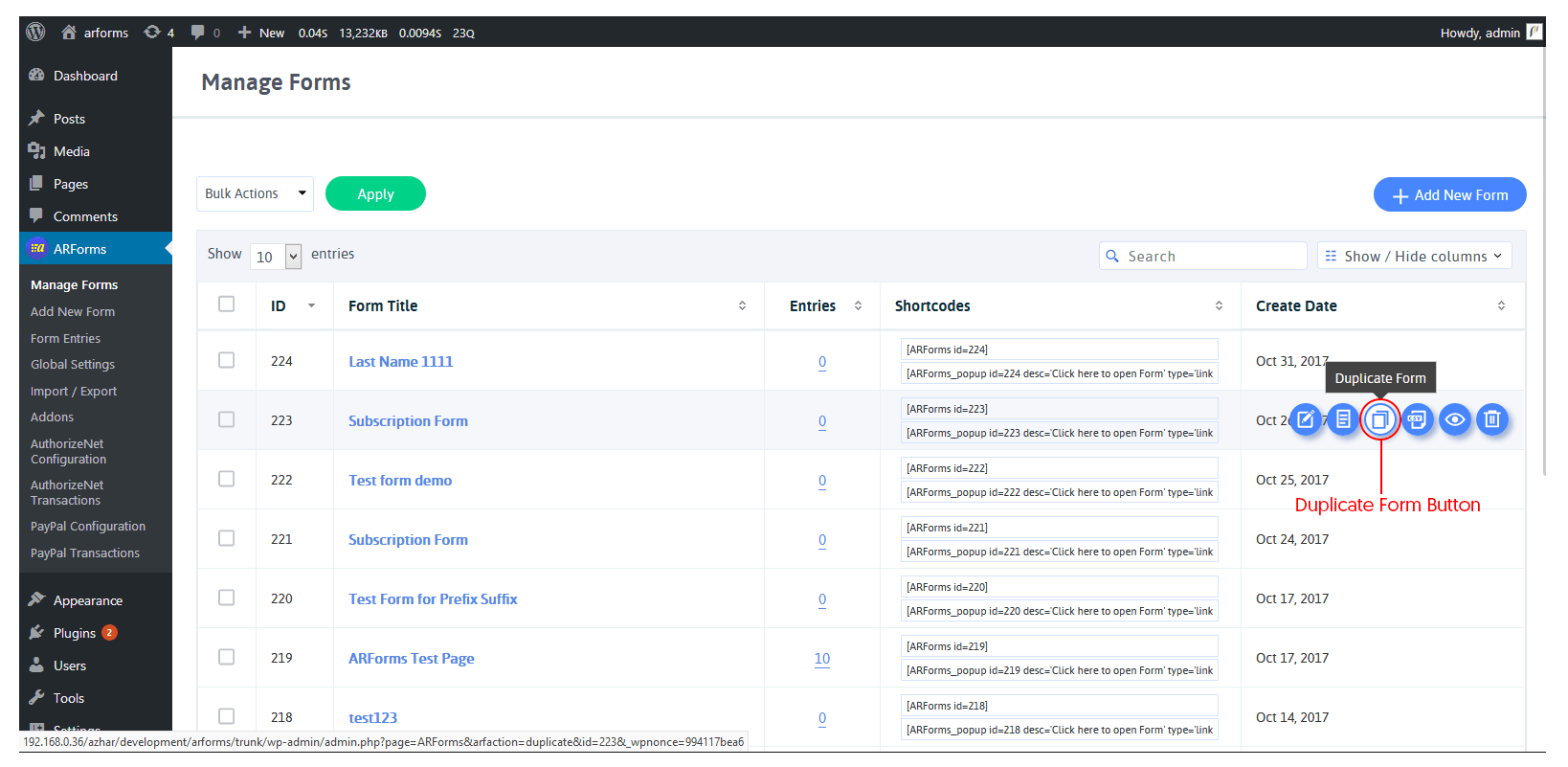The left side of the image features a vertical black rectangle that contains a series of labeled subcategories in white text. These subcategories include "Media," "Pages," and "Comments." Below these in a blue rectangle, more white text is visible. Further down the list, you see options such as "Manage Forums," "Global Settings," "Appearance," and "Plugins," the latter marked with an orange circle. Continuing further down, there are also options for "Users" and "Tools."

On the right side within a white box, the caption "Manage Forms" is displayed. Directly below this caption, there's a green circle containing the word "Apply." At the top right corner, a blue circle with the text "Add New Form" is visible. Moving downward from the form title section, there are various form entries such as "Last Name," "Subscription Forum," "Test Forum," "Subscription Form," and "Test Page." Over to the extreme right, a red circle is connected by a line leading downward to red text that says "Duplicate Form Button."